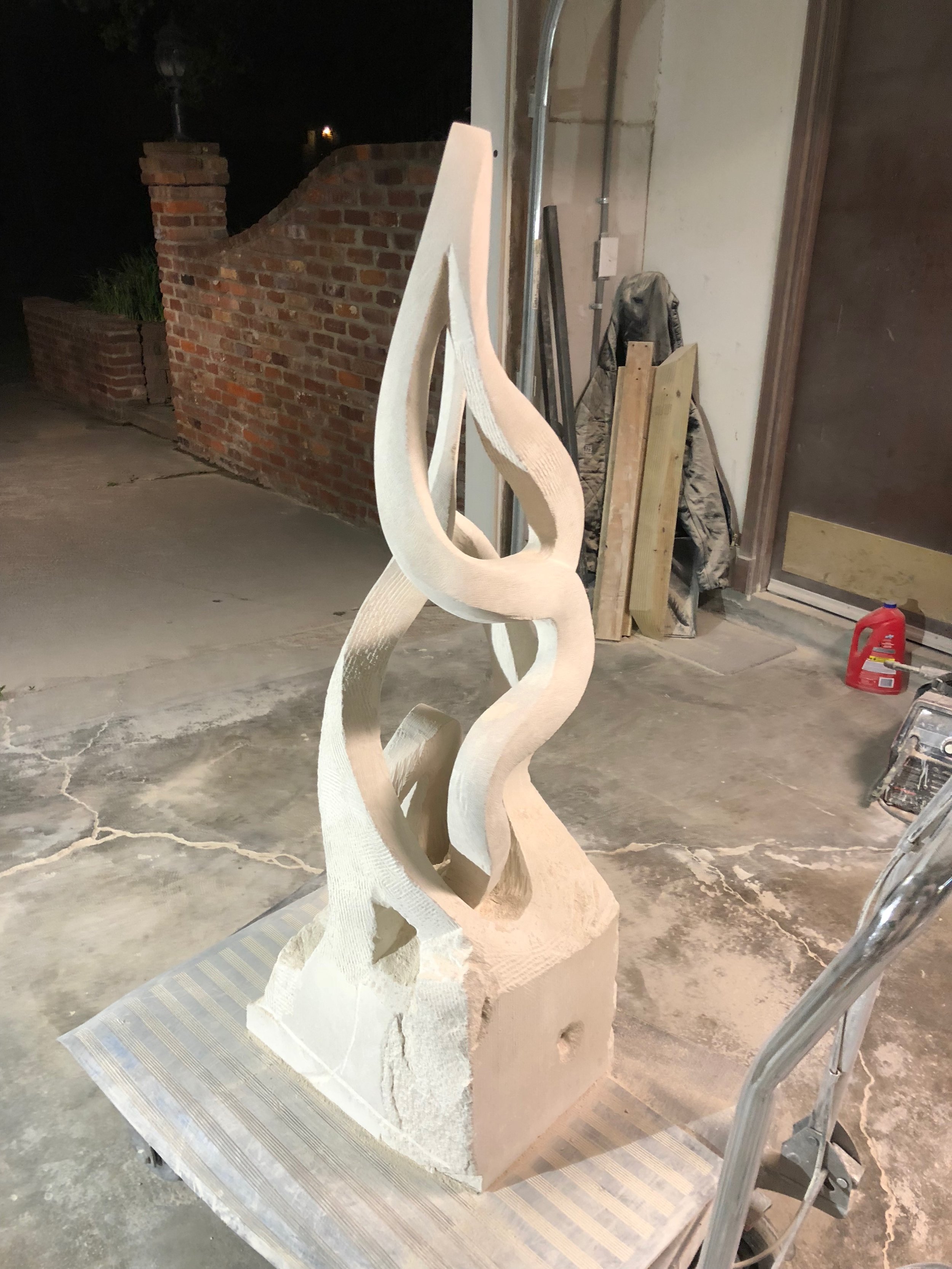This image captures an abstract, unpainted white sculpture that appears to be in the final stages of its creation. The sculpture, reminiscent of twisting branches or a flame, ascends gracefully with elongated lines converging to a point after a series of intricate twists in the middle. It's supported by a striped metal base and stands on a cracked and dusty concrete floor, suggesting recent chiseling work. The setting is an outdoor area that looks like it might be someone's garage or workshop, evidenced by the scattered clay residue, a red jug, a coat hanging near a tall lamp on a brick wall, and various pieces of wood. In the foreground, there is a silver pipe or railing, while the background reveals a brick fence with a gate, giving a sense of depth to the space. The overall ambiance is one of a creative yet gritty workspace, likely under the cover of night.